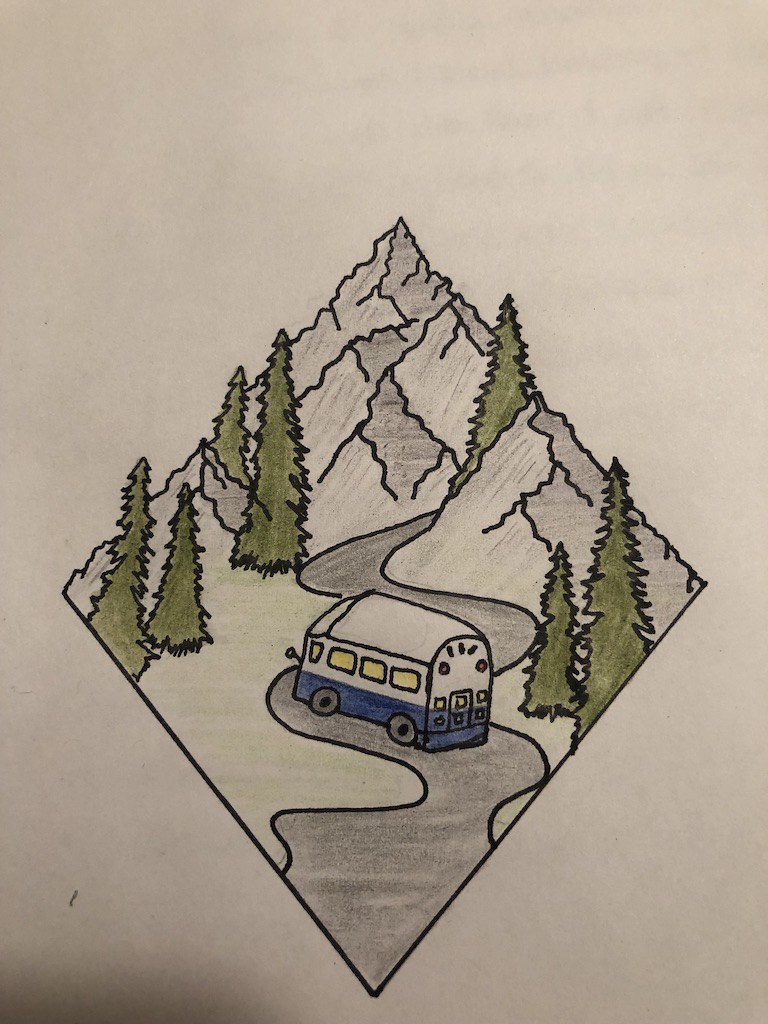This detailed, hand-drawn illustration, created with colored pencils and charcoal on a white background, features a diamond-shaped composition. At the apex of the diamond, rugged mountains capped with snow crown the scene, with tall, slender pine trees sprouting from various points in the rocky terrain. Descending from the peaks, a winding S-shaped road, delineated in dark gray to black with a grassy green perimeter, traverses the entire diamond shape. Along this serpentine road, a small bus, characterized by a white top half, blue bottom half, yellow side windows, and two visible black wheels, makes its journey. The road and surrounding green field are dotted with seven tall, skinny pine trees of varying sizes. This harmonious blend of elements, encapsulated within a rhombus balanced on its point, forms a captivating scene of nature and travel.